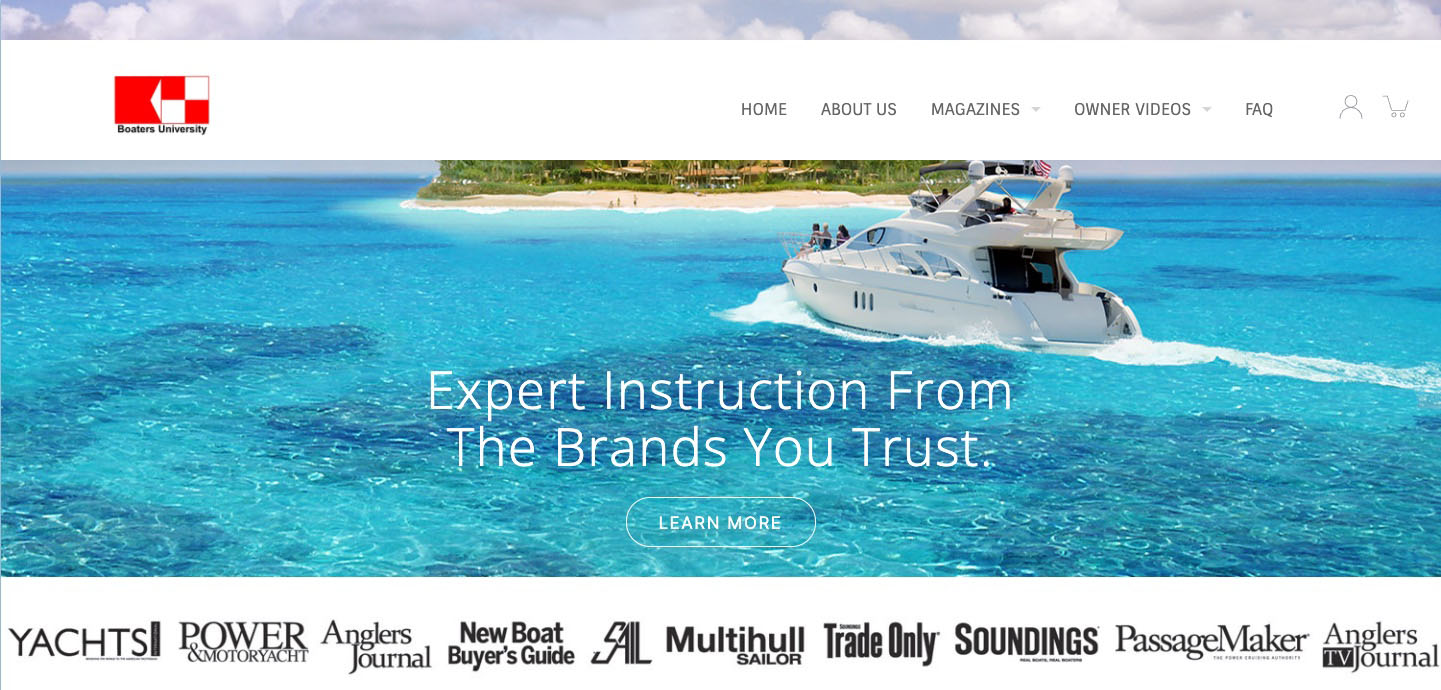In the image, the background showcases the stunningly clear, azure waters of a serene ocean, so transparent that the sandy seabed is visible. Further back, the scene transitions to a picturesque coastline adorned with lush green trees and the rooftops of quaint huts or houses. The focal point of the image is the pristine, tropical blue water.

A sleek, white boat is anchored on the water, with a person seated on the top level and several others gathered at the front gazing out across the horizon. The boat exudes elegance, underscoring the luxurious experience it offers. 

Overlaying this scenic view, text in the lower region of the image reads, “Expert instruction from the brands you trust,” with an option to click and learn more. In the upper left corner, there is a distinctive red and white checkered square. To the upper right, navigation options include Home, About Us, Magazines, Owner Videos, and FAQ.

Positioned beneath the water image are labels in black text, listing various categories: Yachts, Power and Motor Yacht, Angler's Journal, New Boat Buyer's Guide, Multi-Hulled Sailor, Trade Only, Soundings, Passage Maker, and Angler's TV Journal.